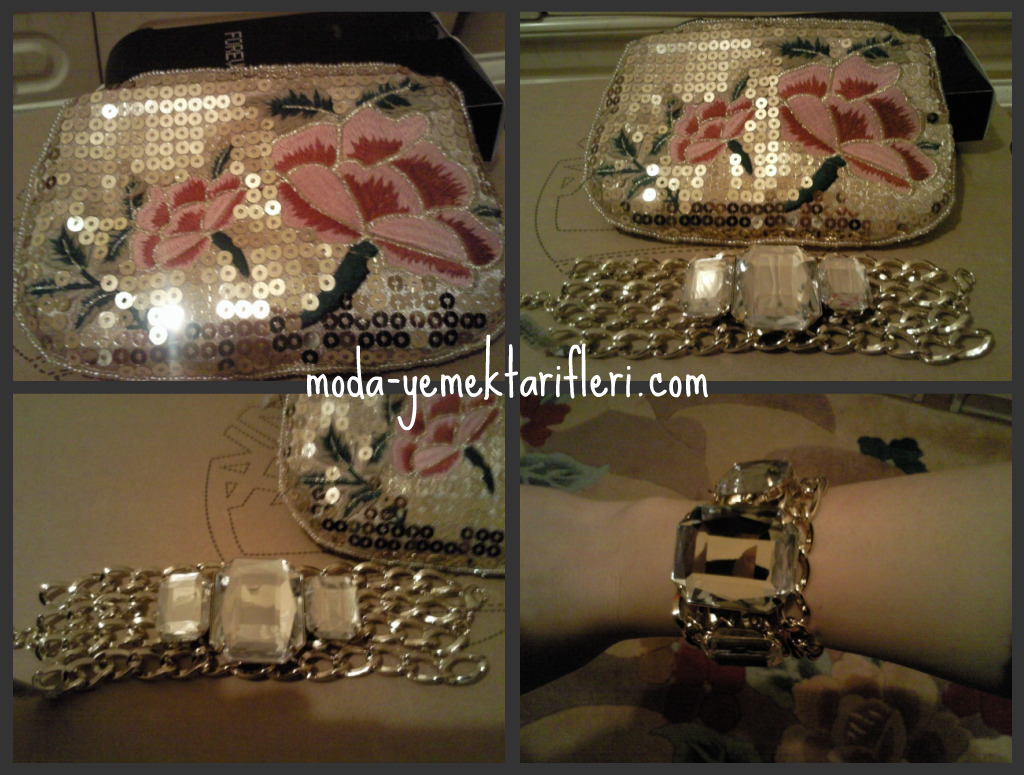This advertisement for Moda Yemak Tarifleri.com is divided into four distinct, equally-sized sections, each framed with a thin gray border, showcasing various accessories. The top left image features a detailed shot of a small, sequin handbag in gold, adorned with green stems and two pink roses, one tilted left and the other right. Behind the purse, partially visible black text reads "FOREU." The top right image displays the same sequin purse paired with a bejeweled metal bracelet, prominently featuring large, faux quartz crystals set in a gold band. The bottom left section offers a close-up of the bracelet, emphasizing its rectangular sections studded with diamond-like jewels. The lower right quadrant shows the bracelet in use, elegantly draped around a woman's wrist. At the center of the advertisement, the brand's website, Moda Yemak Tarifleri.com, is written in stylish white text.